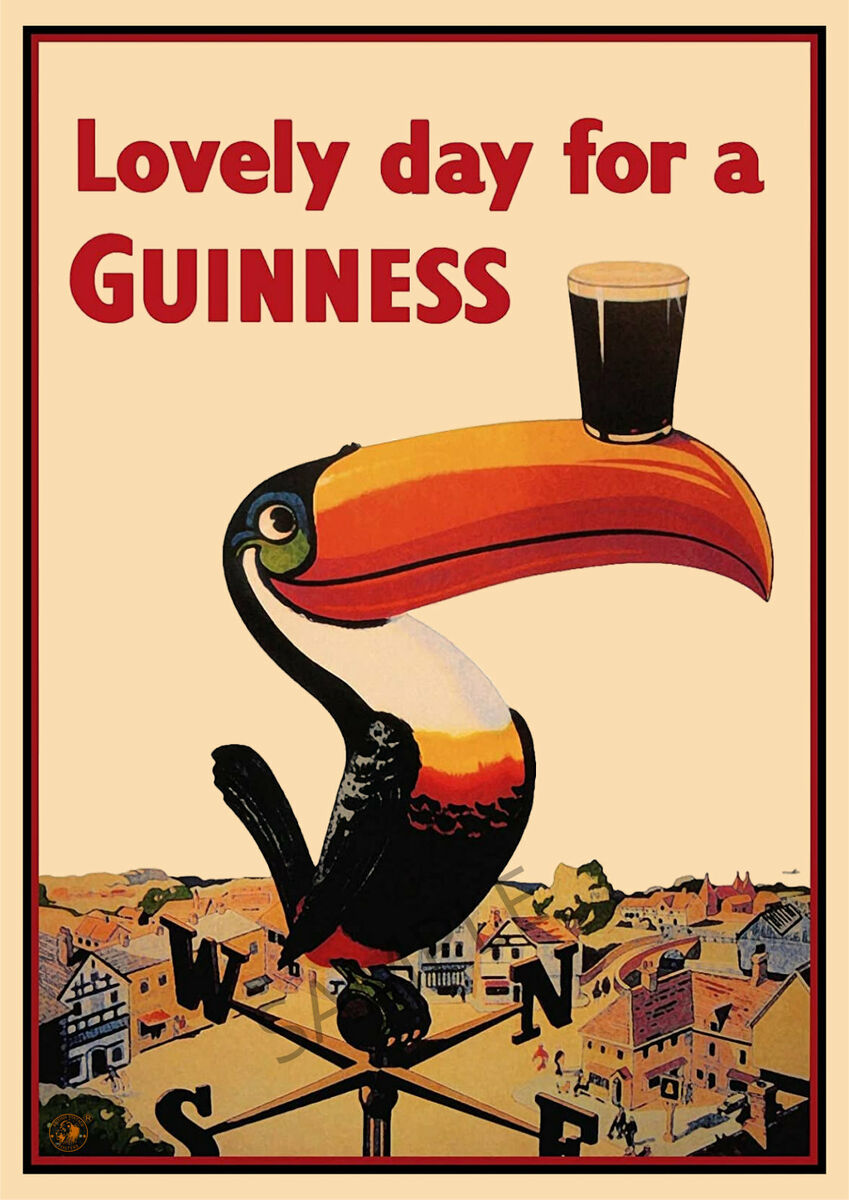This detailed poster advertisement for Guinness beer showcases a whimsical, colorful toucan perched atop a weather vane. The poster has a cream beige background, bordered by a black frame with a red inner line. At the top, bold red text declares, "Lovely Day for a Guinness." The vibrant cartoon-like toucan, depicted with an array of colors including black, white, yellow, orange, and green, sports a cheerful expression. A notable feature is his large orange beak, which bears a glass of dark, foaming Guinness beer. The weather vane beneath the toucan prominently displays the cardinal directions N, S, E, and W. Below the weather vane, a quaint, cartoonish representation of a village is visible. The overall composition creates a charming and inviting scene that highlights the toucan and the Guinness beer.